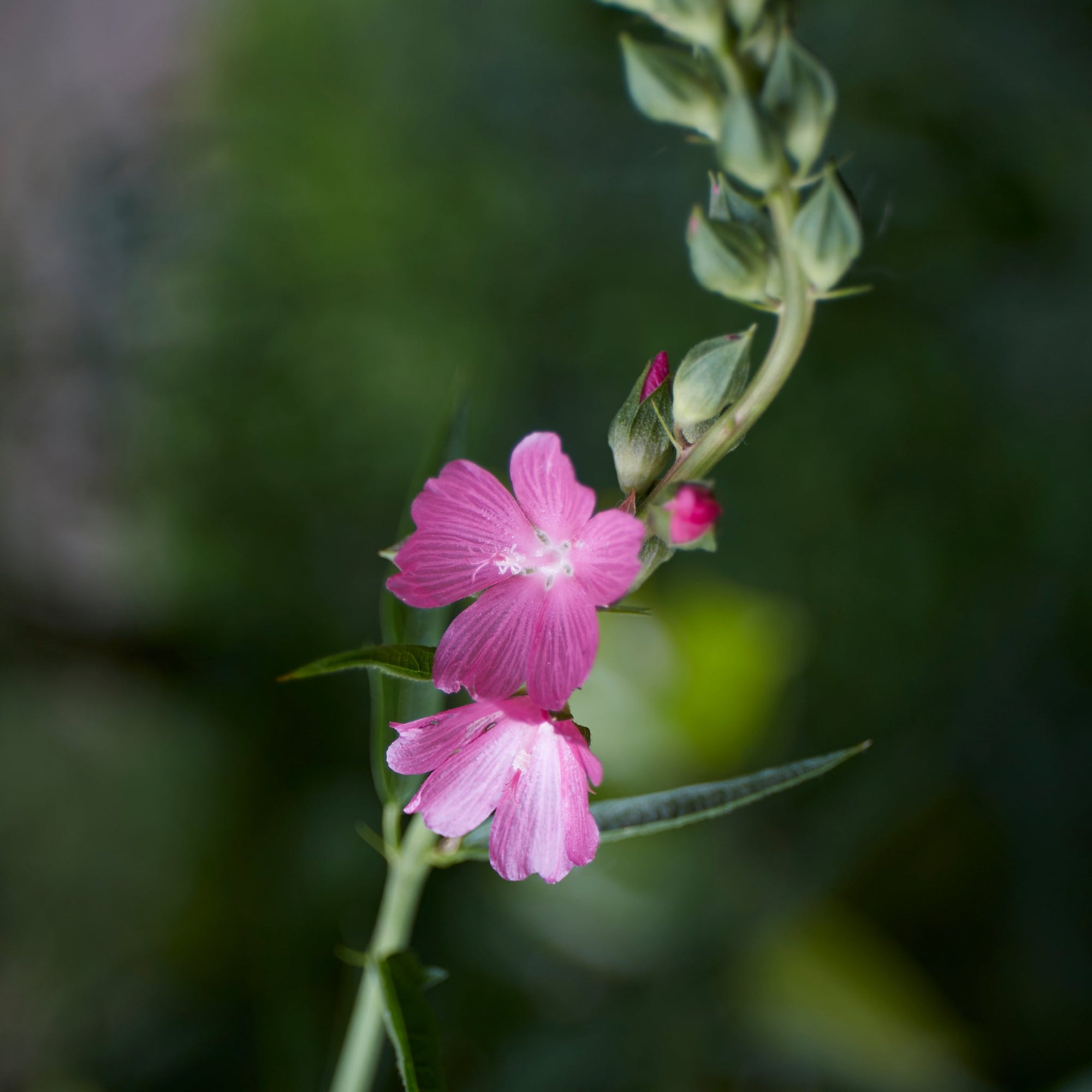The image features a beautifully detailed close-up portrait of a flower with vibrant pink petals that appear freshly bloomed. The flower's stem is a rich green, adorned with straight leaves that add texture to the composition. At the center of the photo, the main flower stands out with its partially open petals, displaying shades of pink, white, and lighter green. Above this central flower, a secondary stem rises, leading to a cluster of at least six buds. Most of these buds are closed, though two near the central flower begin to reveal hints of pink. The background is artistically blurred, transitioning from light blue on the left to green on the right, making the flower and its vibrant colors pop prominently in the foreground. The entire scene is free of any text, allowing the natural beauty of the flower to captivate the viewer's attention fully.